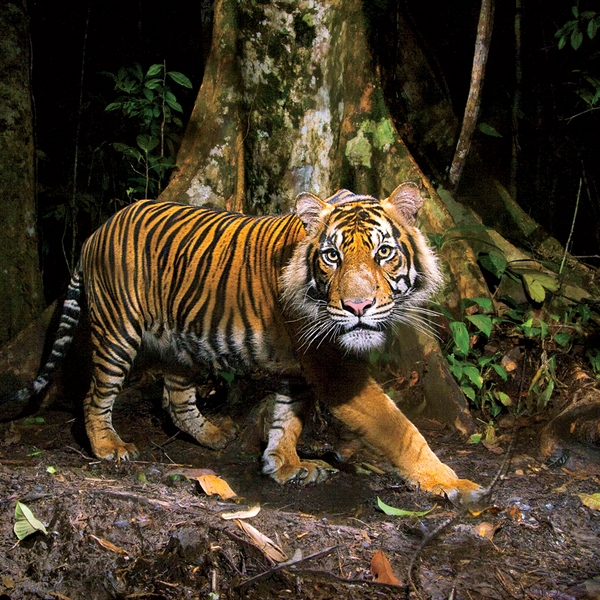This is a photograph of a tiger in a forest at nighttime. The tiger's body is a striking blend of yellow with black stripes, providing a captivating contrast. In this side view, the tiger's head is turned towards the viewers, creating an engaging and direct gaze. Its face showcases a combination of yellow, black, and white hues, with light pink ears and a pink nose, complemented by noticeable whiskers near the nose. The scene includes a tree trunk behind the tiger, surrounded by small plants and shrouded in the darkness of the forest. The ground beneath is brown from the soil, with visible patches of wetness, indicating it might have rained recently. The composition captures the tiger centered in a square frame, appearing both majestic and slightly surreal, as if teetering between an actual photograph and a digitally created image.